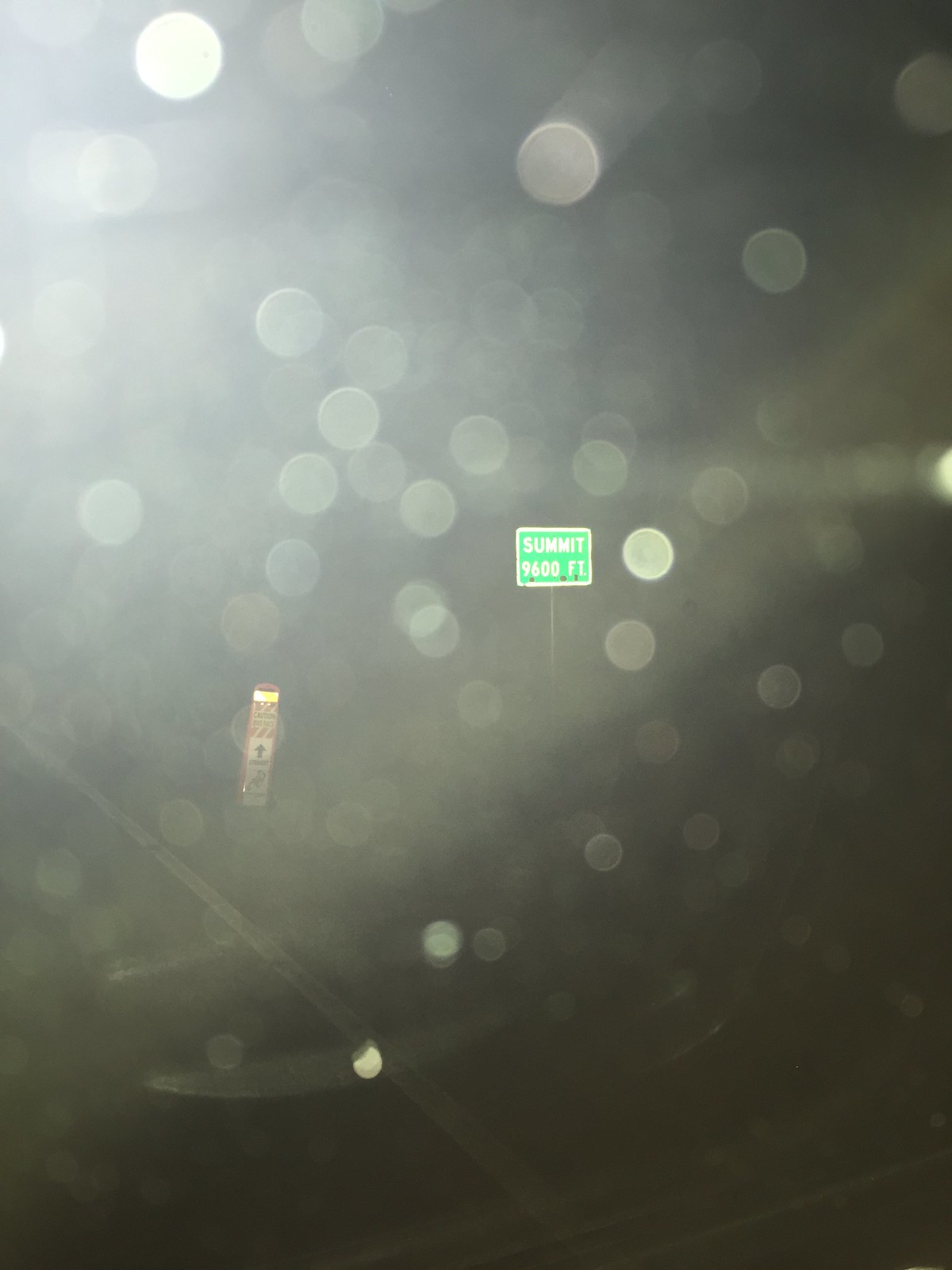The photograph is an extremely blurry image taken at night, characterized by a dark gray, almost black background adorned with numerous small, white orbs floating across the scene, which might indicate light refraction or a blurred camera lens. Dominating the center of the image is a green street sign with a white border and white text that reads "SUMMIT 9600 FT." The sign is brightly lit against the dark backdrop, making it the most distinguishable element in the photo. To the left and slightly below the sign, there appears to be a tall, rectangular object with a reddish-orange hue, possibly a mile marker or roadside post. In the foreground, faint outlines suggest the presence of paved ground and perhaps train tracks, though the overall blurriness makes these details difficult to ascertain clearly.